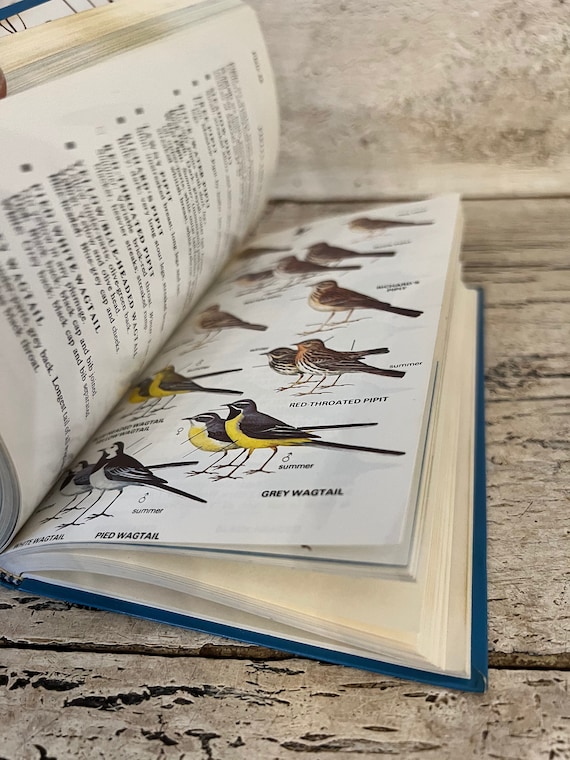This image showcases an open book lying on a worn, dark tan wooden surface, resembling an aged wooden bench or box. The book, with a dark blue hardcover, is opened to a middle page, revealing detailed, hand-drawn illustrations of various birds on the right-hand page. These birds are depicted in diverse colors such as black and white, yellow and black, and shades of orange and brown, and include specific species like the pied wagtail, gray wagtail, and red-throated pipit. The left page, oriented vertically, contains blurred text which likely describes the birds illustrated on the adjacent page. The readable labels beside the bird illustrations include the word 'wagtail'. The book appears to be a medium-thick physical textbook, emphasizing its focus on ornithology with its informative and visual content.